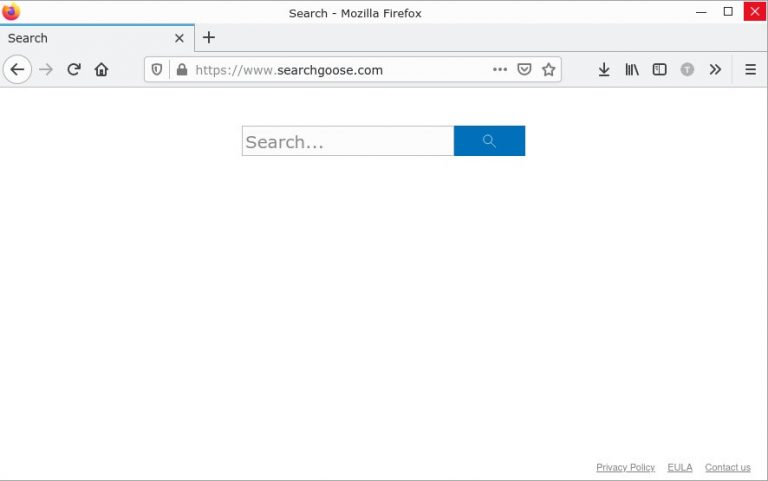This image showcases the Mozilla Firefox browser interface. In the upper-right corner, there are three buttons: the white "X" close button enclosed in a red box, the middle maximize button, and the minimize button. Centrally located, you can see the text "Search Mozilla Firefox," sitting prominently at the top-center of the window. On the upper-left corner is the identifiable Firefox logo.

Beneath the logo, there is an active tab with a title indicating ongoing search activities. Each tab has its own close button marked with an "X." Just below this tab, the classic browser navigation elements are visible: the back arrow, the forward arrow, the refresh button, and the home button.

Within the address bar, the text "www.searchgoose.com" is displayed. Below this are several spaces, leading to the main section of the browser window. Here, a primary search bar is featured, accompanied by a blue search button, hinting at the current functionality available to the user on this particular webpage.